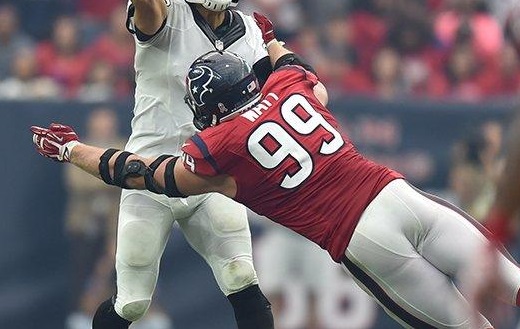This image captures an intense moment during a football game, focusing on two players in action. The background is blurry, with indistinct stands, fans, some dressed in red, and a black wall dividing the spectators from the field. In the foreground, player in a white jersey and white pants stands facing the action, with his right arm cut off just above the elbow at the top of the image. His left leg is forward, and his feet, clad in black socks, are cut off just below the knees. Opposite him is player number 99, wearing a red jersey with white lettering and white pants, along with a Houston Texans helmet and red gloves. This player is mid-air, angled downward as if leaping or tackling, with outstretched arms and his body extending off the frame at the bottom right corner. Both players are visibly wearing padding for protection.